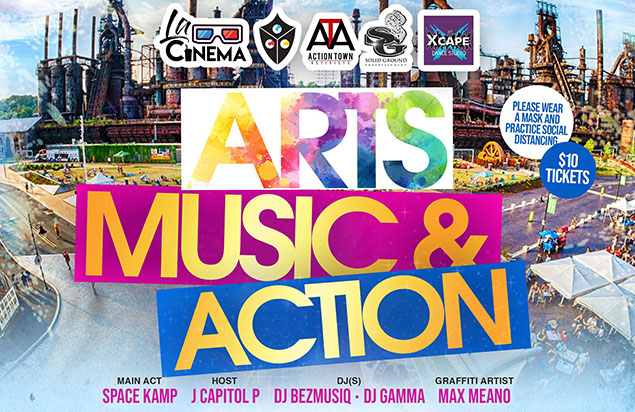Poster for "The Cinema Presents: Arts, Music, and Action Event"

This vividly detailed poster promotes an eclectic event combining arts, music, and action, though it notably lacks specifics on the location and date. The background features a bustling cityscape with industrial elements like refineries and smokestacks, adding an intriguing juxtaposition to the cultural activities advertised. 

At the top of the poster, "The Cinema" is prominently displayed alongside small icons such as a shield, "ATA Action Town," a sound-related icon, and a purple icon labeled "X Cape." Central to the design, the word "Arts" stands out in a striking rainbow ombre font on a white bar, followed by a pink bar with gold letters that read "Music And," and a blue bar with gold letters that proclaim "Action." 

The bottom section provides details about the event's main attractions: "Main Act: Space Camp," alongside performances by "Host JP," DJs "Biz Muke" and "Gamma," and a graffiti display by artist "Max Minow." Additionally, the poster encourages attendees to wear masks and practice social distancing, with tickets priced at ten dollars. The visual depiction includes various fairground elements such as tents and awnings, suggesting an outdoor setting anticipated to draw a significant crowd. Despite the lack of specific logistical information, the vibrant and elaborate design underscores the multidisciplinary offerings of this intriguing event.